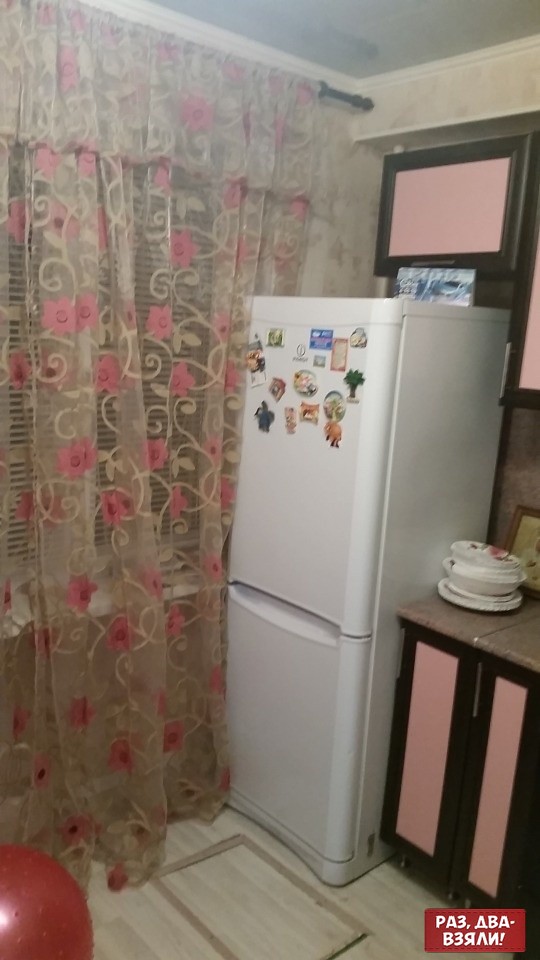This detailed, indoor color photograph captures an outdated kitchen in need of repair. The focal point is a slim, white refrigerator-freezer with magnets affixed to its top section, positioned slightly off-center to the right. The kitchen floor appears to be white linoleum or tiles with light grout lines, possibly featuring a small trap door. Adjacent to the refrigerator are pink cabinets with a black border, topped with a marble-like countertop cluttered with a miscellaneous stack of dishes, bowls, and plates.

To the left of the refrigerator is a window, adorned with semi-transparent curtains draped from a black curtain rod spanning floor-to-ceiling. These sheer curtains are decorated with pink roses and white squiggly lines or vines. Above and around the refrigerator is additional cabinetry with pink panels and dark brown or black frames, matching the lower cabinets.

The walls of the kitchen are painted a light salmon pink or greyish cream color, with a white ceiling overhead. In the bottom right corner of the image, there is a red rectangle label featuring Cyrillic writing, reading "PA3ABA B3 хэрэглээ exclamation mark". Additionally, a partially visible red disc or semicircle is noted in the bottom left corner of the photograph. An orange ball is also visible on the floor, adding a touch of unexpected color to the scene.